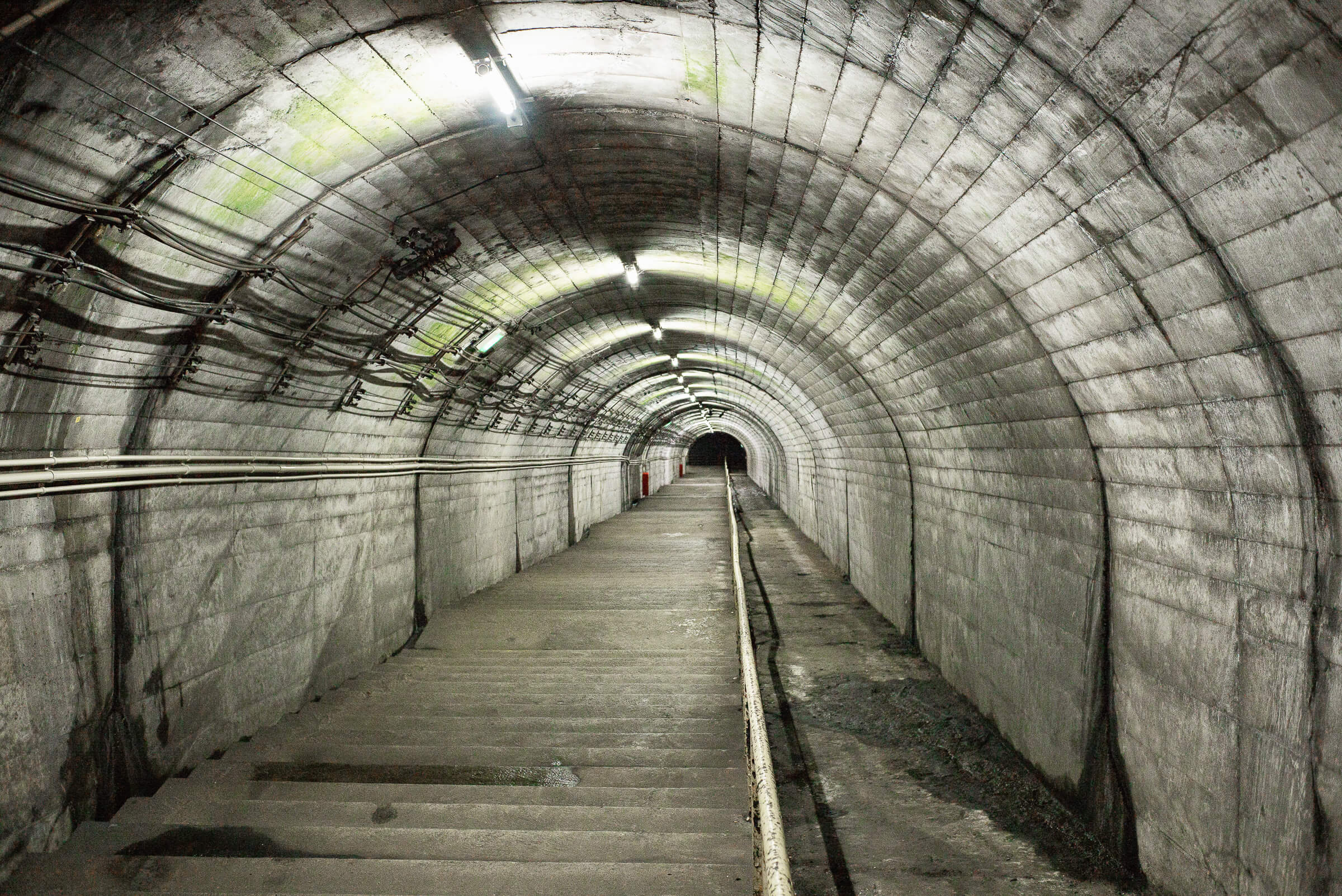This photograph captures an indoor, underground tunnel. The tunnel, constructed from gray cement, features a curved, round ceiling lined with white tiles that are streaked with shades of gray, green, and yellow. Lighting fixtures are evenly spaced along the ceiling, casting a bright glow throughout the damp and humid environment. On the left side of the tunnel, rows of piping and wiring run along the wall, emphasizing the tunnel's engineered function. Below, gray concrete steps, some seemingly damp with darkened spots, descend into the depths of the tunnel. A white metal barrier separates these steps from a rougher, stony area to the right, which likely serves as a drainage channel for water runoff. The photograph conveys a sense of an endless, narrow passageway leading into the darkness, enriched with details of its industrial and utilitarian design.